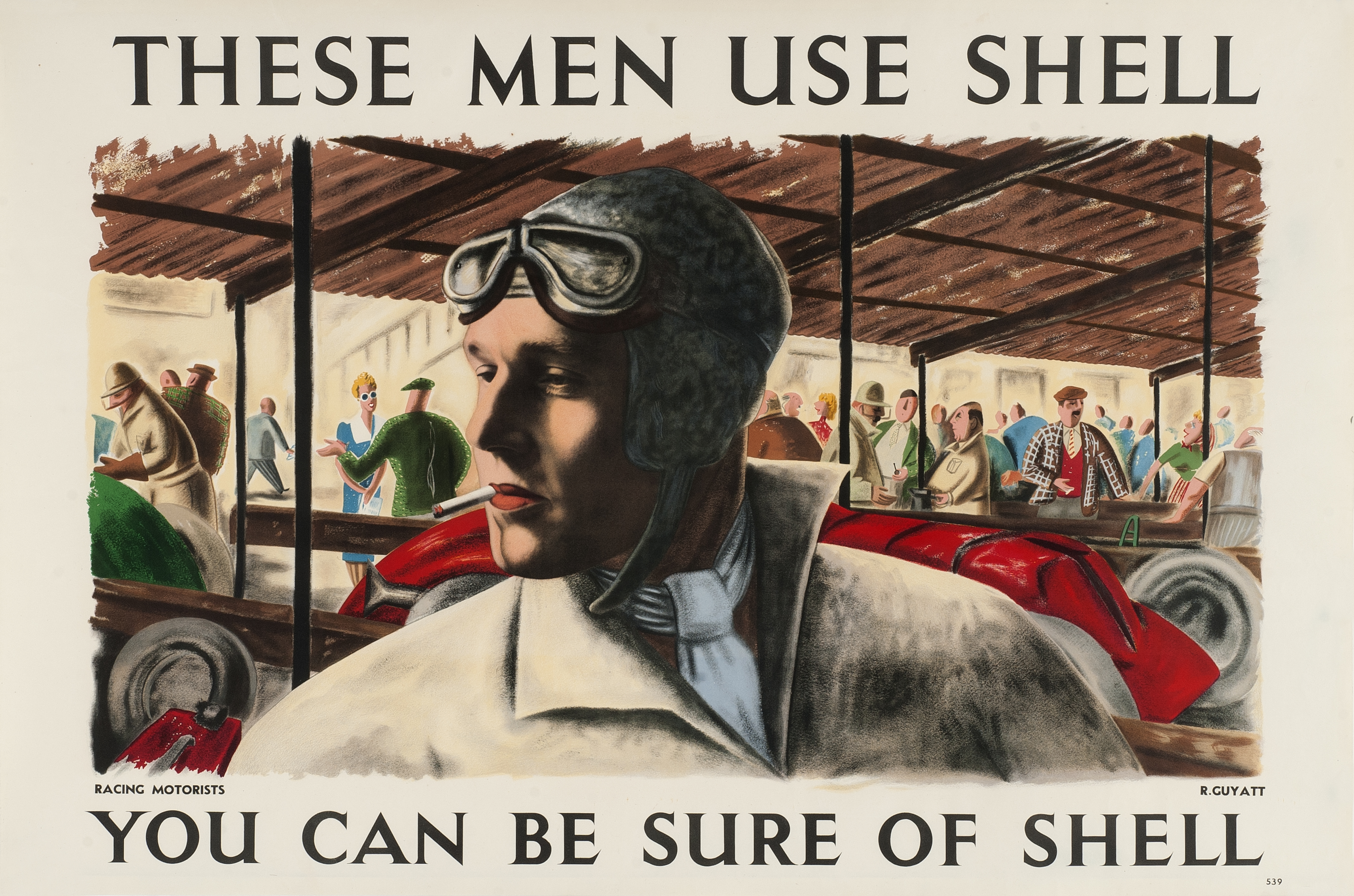This vintage advertisement features a colorful illustration typical of the 1930s or 40s, set within a gray-bordered, vertically oriented frame. At the top, bold block letters declare, "THESE MEN USE SHELL," while the bottom of the poster confidently asserts, "You can be sure of Shell." Dominating the center is a painting of a classic race car driver. He wears an old-style leather racing helmet, with goggles perched on his forehead, and sports a white scarf tied around his neck, adding a touch of flair to his grayish-beige coat. A cigarette dangles from his mouth as he gazes to his right, his body facing forward in a relaxed posture, suggesting he has just finished racing. Behind him, a red race car is partially visible, complemented by other race-track elements such as a car wheel over his right shoulder. In the far background, a bustling scene unfolds with people engaged in various activities, possibly selling concessions or simply conversing under a corrugated or wooden roof structure. Tiny letters at the lower left of the painting read "Racing Motorist," adding authenticity to the scene. These details cohesively capture the atmosphere of an old-timey race track, highlighting the allure and prestige associated with Shell products.